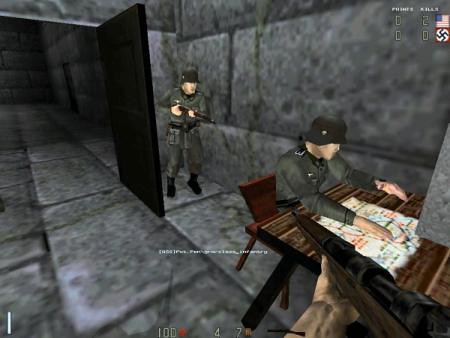Screenshot of a tense standoff in a video game: Inside a cement-walled building featuring alternating light and dark gray blocks, two soldiers confront each other. On the left side, an open black door reveals a soldier in a light gray uniform holding a shotgun aimed at another soldier. The second soldier, seated at a desk and focused on a piece of paper, seems oblivious to the immediate threat. In the bottom right corner, a portion of another character appears, also wielding a shotgun pointed at the first soldier hidden behind the door. The scene encapsulates a complex and suspenseful moment within the game, highlighting the players' tactical positioning and imminent action.